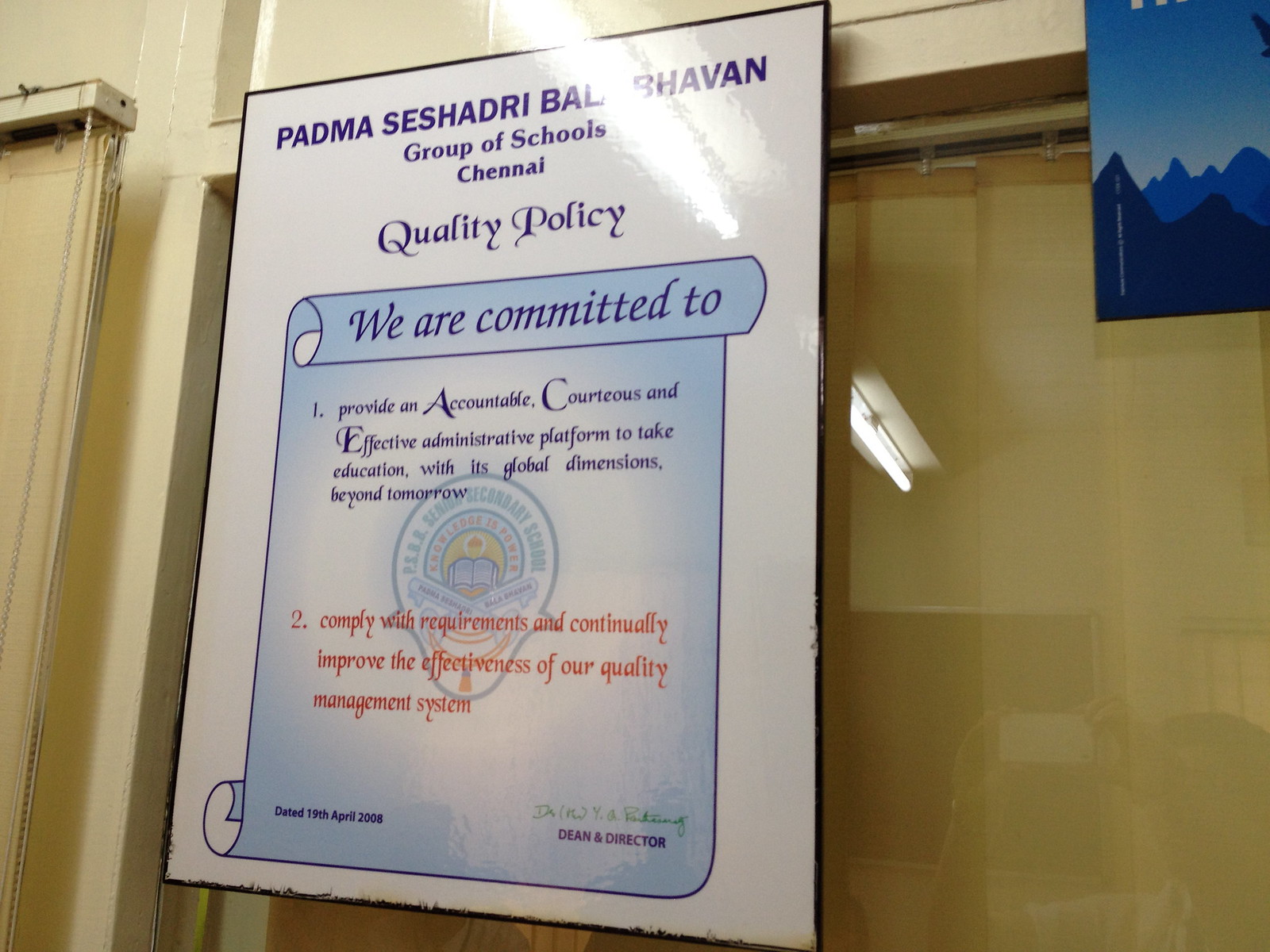The image features a white framed plaque mounted on a tan wall, viewed diagonally from the right side. In the top right corner of the image, a poster displaying jagged blue mountains can be seen. 

The plaque itself is illuminated by a rectangular light hanging above, creating a reflection that partially obscures the text. At the top of the plaque, in all capitalized dark blue text, it reads "PADMA SESHADRI BAL BHAVAN." Below this, in title case, it states "Group of Schools."

The main text of the plaque is titled "Quality Policy" in a fancy script-like font. It begins with a statement on a blue scroll that reads, "We are committed to," followed by two points: "Provide an accountable, courteous, and effective administrative platform to take education with its global dimensions beyond tomorrow" written in blue, and "To comply with requirements and continually improve the effectiveness of our control management system" written in red.

Towards the bottom of the plaque, there is an icon resembling a book encircled by a yellow aura, representing an award. The plaque is signed by the Dean and Director, dated from 2008.